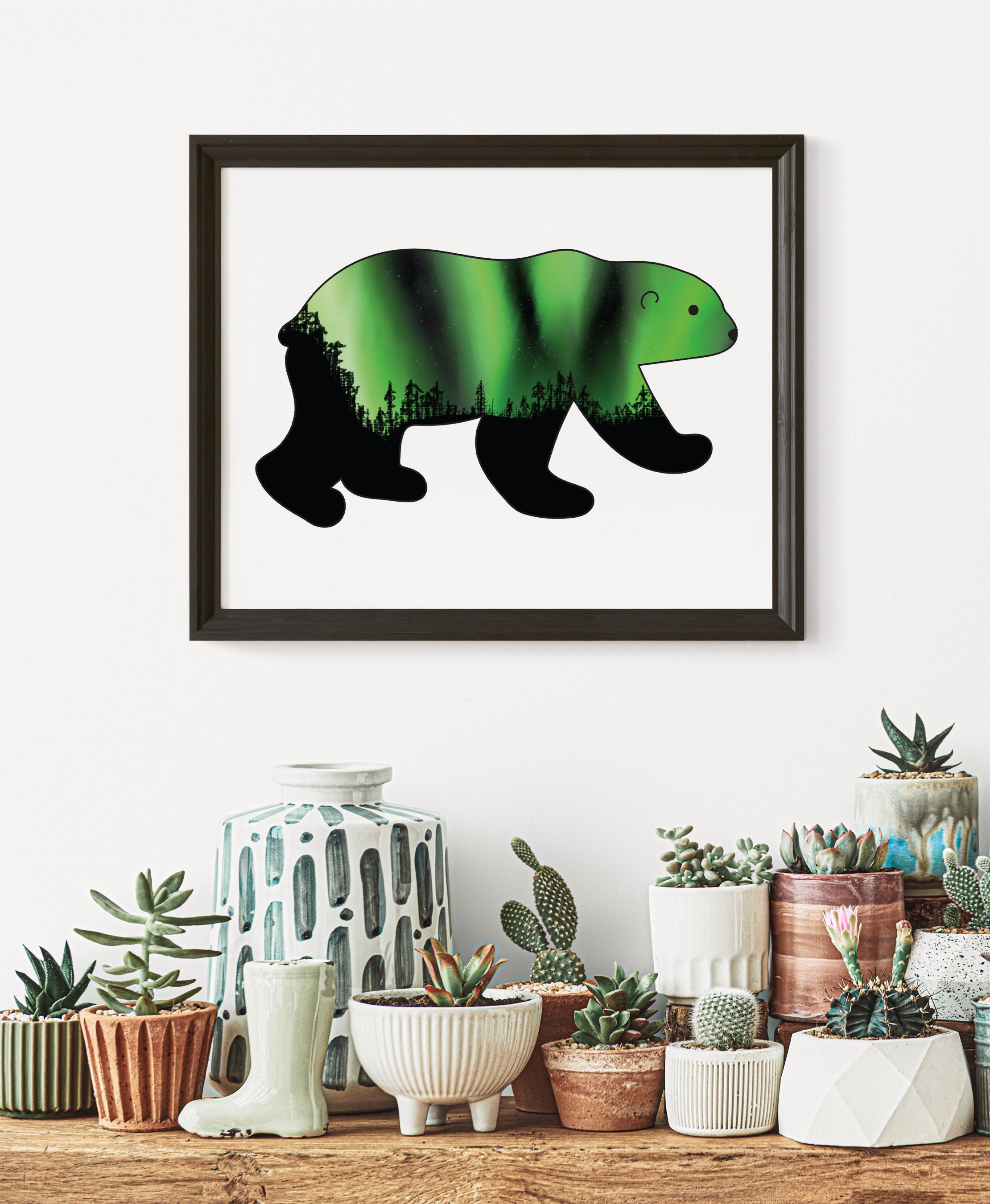In this photo, we see a living room with a white wall adorned by a black-framed painting of a unique bear. The bear's body features a lime green upper portion, resembling the northern lights illuminating a forest, and black legs. The painting serves as a vivid central piece in the room. Below the painting, on a light brown wooden shelf or tabletop, numerous small planters are neatly arranged. These planters host various cacti and succulents, adding a touch of greenery to the space. The planters include a mix of colors and designs: a small green planter with a succulent, a brown planter with a taller succulent, a white figurine in the shape of a mud boot, a large white vase decorated with green cucumbers, and several white, terracotta, and orange planters each containing a cactus or succulent. One of the planters, a large white vase, stands out as it does not contain any plants. The living room is decorated with numerous other elements, including a variety of bowls, enhancing the cozy yet eclectic atmosphere of the space.